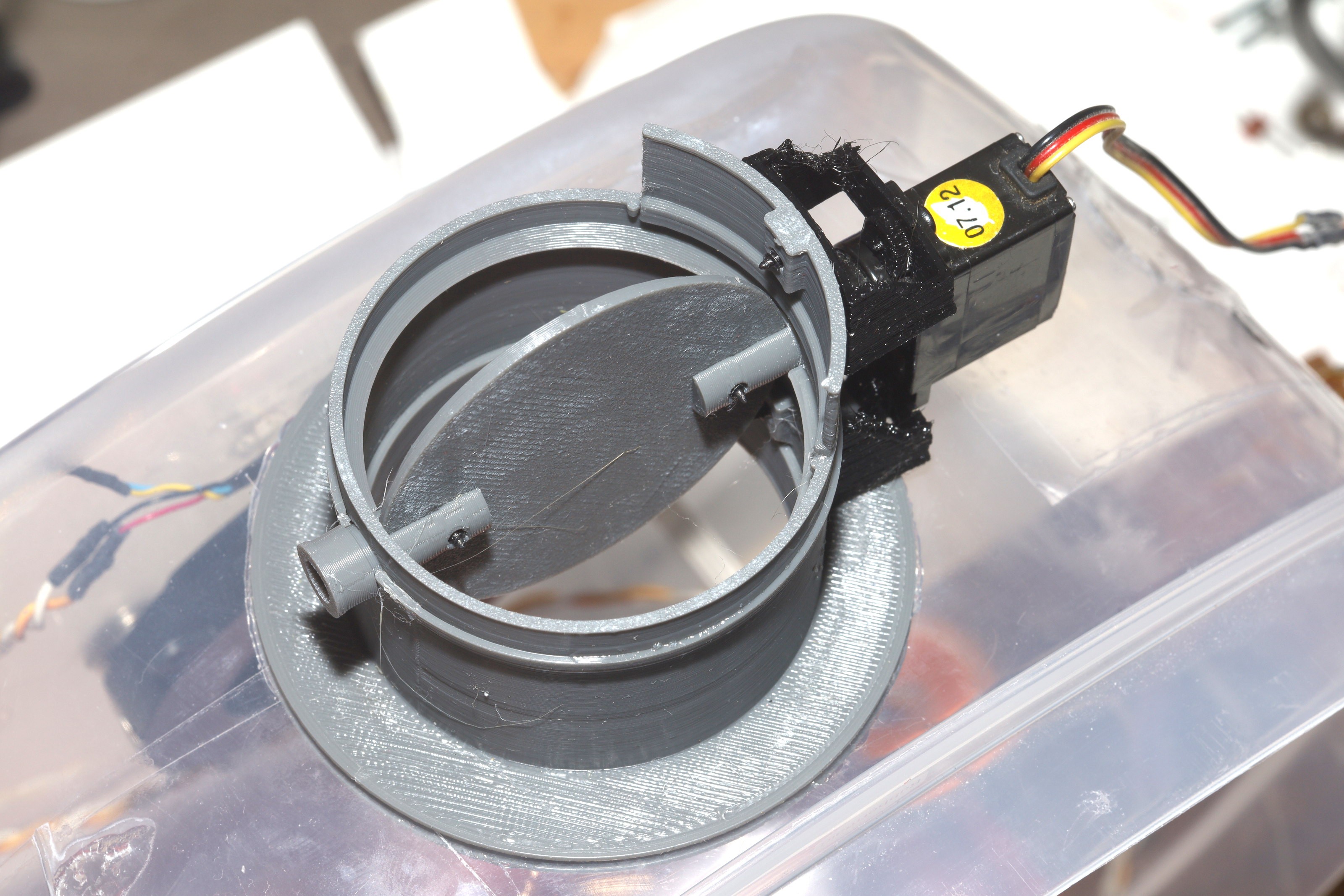This is a highly detailed photograph of an electrical device, prominently featuring a gray cylindrical component, possibly made of painted metal or plastic. The cylinder is notable for housing a circular disc that appears to be suspended within it. Attached to the right side of the cylinder is a black box-like structure, marked with a yellow sticker reading "07.12." Emerging from this black component is a cable composed of red, black, and yellow wires. The entire assembly is situated on top of a clear plastic container filled with other similar components and cables, all set against a bright, illuminated white background. Additional visible elements include another electrical wire inside the container, featuring connections secured by black electrical tape. The image is contemporary in appearance, emphasizing the device's modern and intricate design.